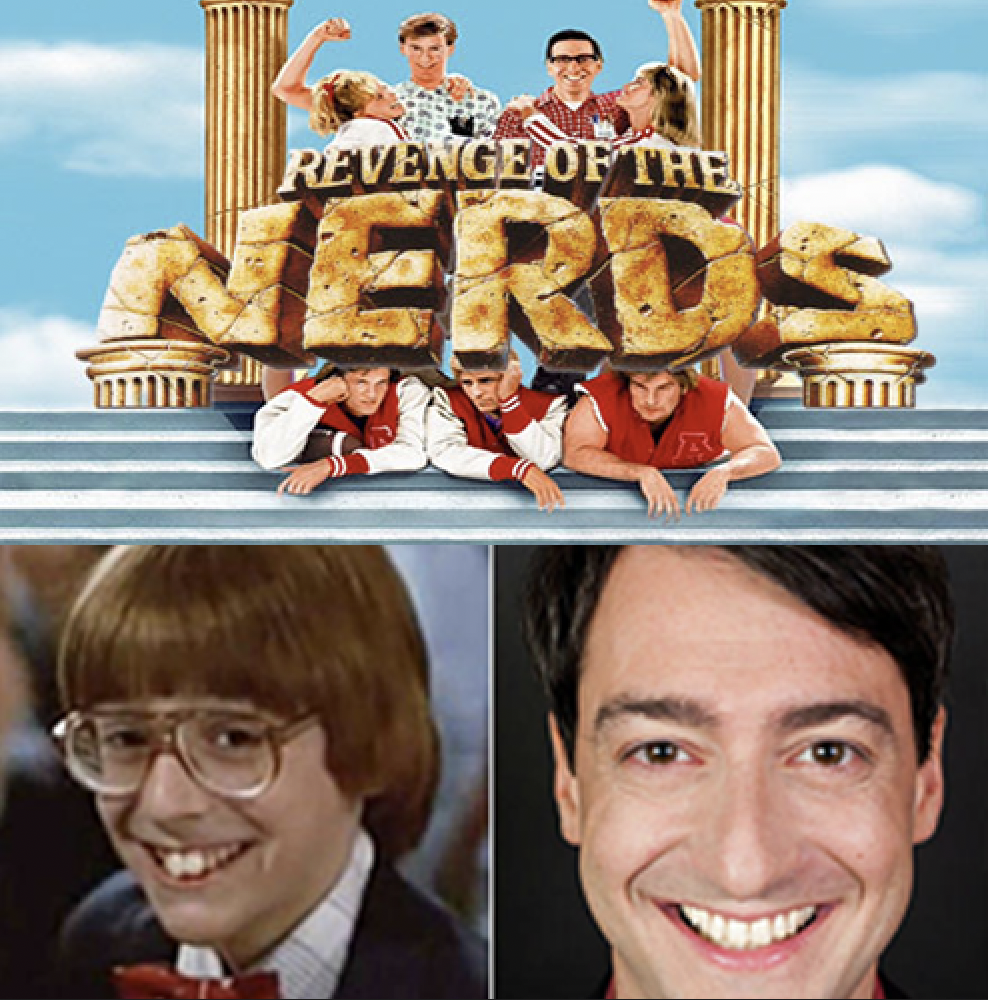The image is an advertisement for the movie *Revenge of the Nerds*, composed of three distinct panels. The upper half of the image is a large rectangular movie poster set against a blue sky backdrop with scattered white clouds. Framing the composition on either side are two Grecian-style tan pillars. In the center of the poster, four characters—two women flanking two men—stand triumphantly with the women embracing the men and smiling up at them. Below this group, the movie title "Revenge of the Nerds" is prominently displayed in gold lettering.

Positioned beneath the lettering on the ground are three men, depicted as fallen jocks, wearing red and white jackets—two in varsity jackets and one in a red life preserver vest. The word "Nerds" appears to be crushing these jocks, emphasizing the nerds' triumph.

The bottom half of the image contains two square panels. The left panel features a younger, nerdy-looking man with red hair styled in a bowl cut. He's wearing large tortoiseshell glasses, a red bow tie, and a black jacket over a white shirt. The right panel showcases the same man, now older, with short black hair parted to one side, smiling directly at the viewer.

This detailed portrayal combines elements from each person's description to provide a comprehensive and vivid caption.